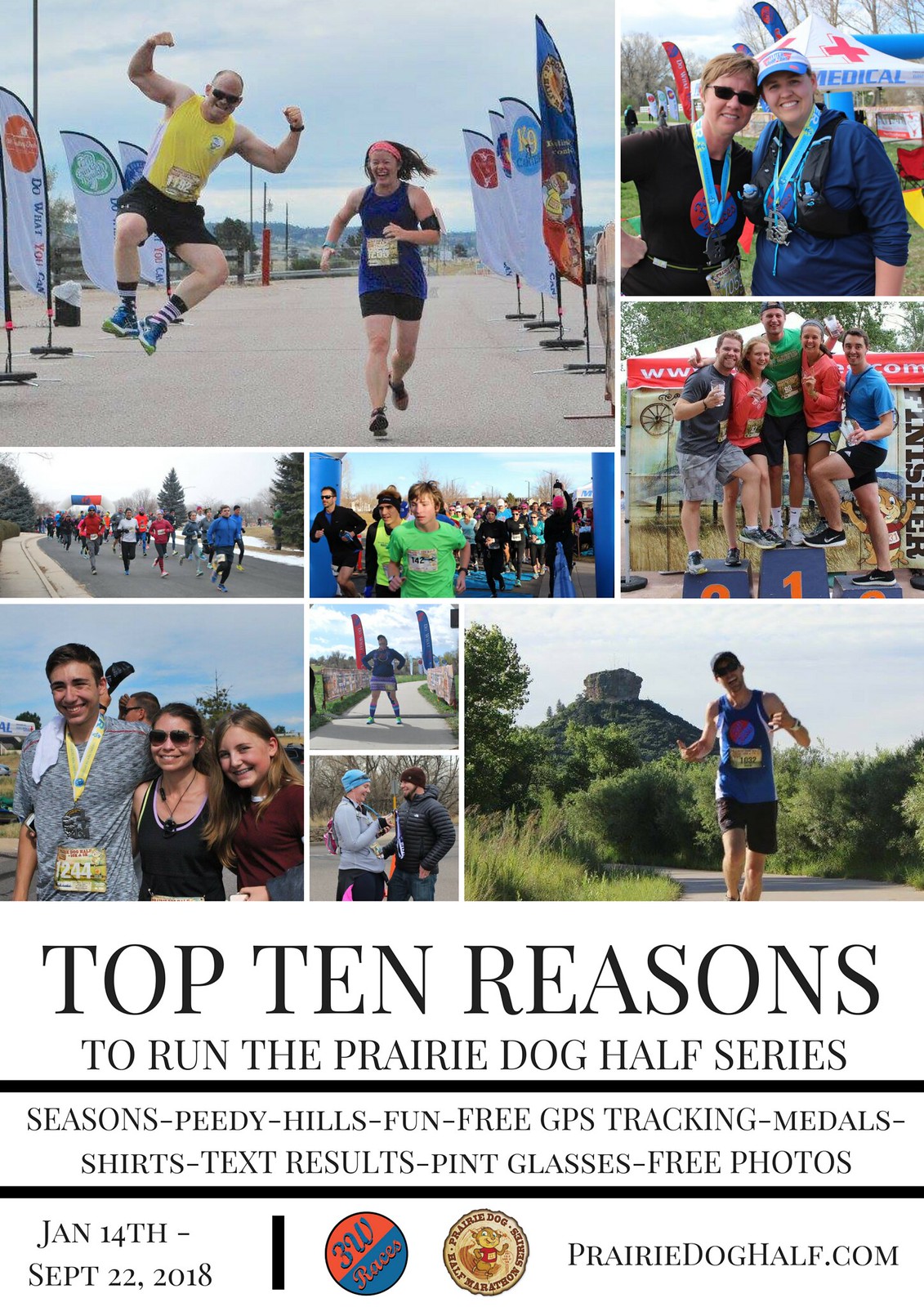This vibrant and energetic poster for the Prairie Dog Half Series features a large collage of nine engaging color photos of runners. The top left image is the most prominent and captures two enthusiastic participants nearing the race finish line, flanked by flags. The woman in a blue tank top and pink bandana, with a race number, races forward with a wide smile, while the man beside her in a yellow tank top and black shorts joyfully flexes his biceps and kicks his heels in the air. Surrounding this are various snapshots of runners proudly displaying their medals, standing on the winners’ podium, and taking post-race photos. 

Below the collage, a white section with black text lists the "Top 10 Reasons to Run the Prairie Dog Half Series": Seasons, PD, Hills, Fun, Free GPS Tracking, Medals, Shirts, Text Results, Pint Glasses, and Free Photos. The bottom left corner features the dates "January 14th - September 22nd, 2018," while the bottom right displays the event website, PrairieDogHalf.com, along with two circular logos. This poster serves as a dynamic and inviting advertisement for the running race series.